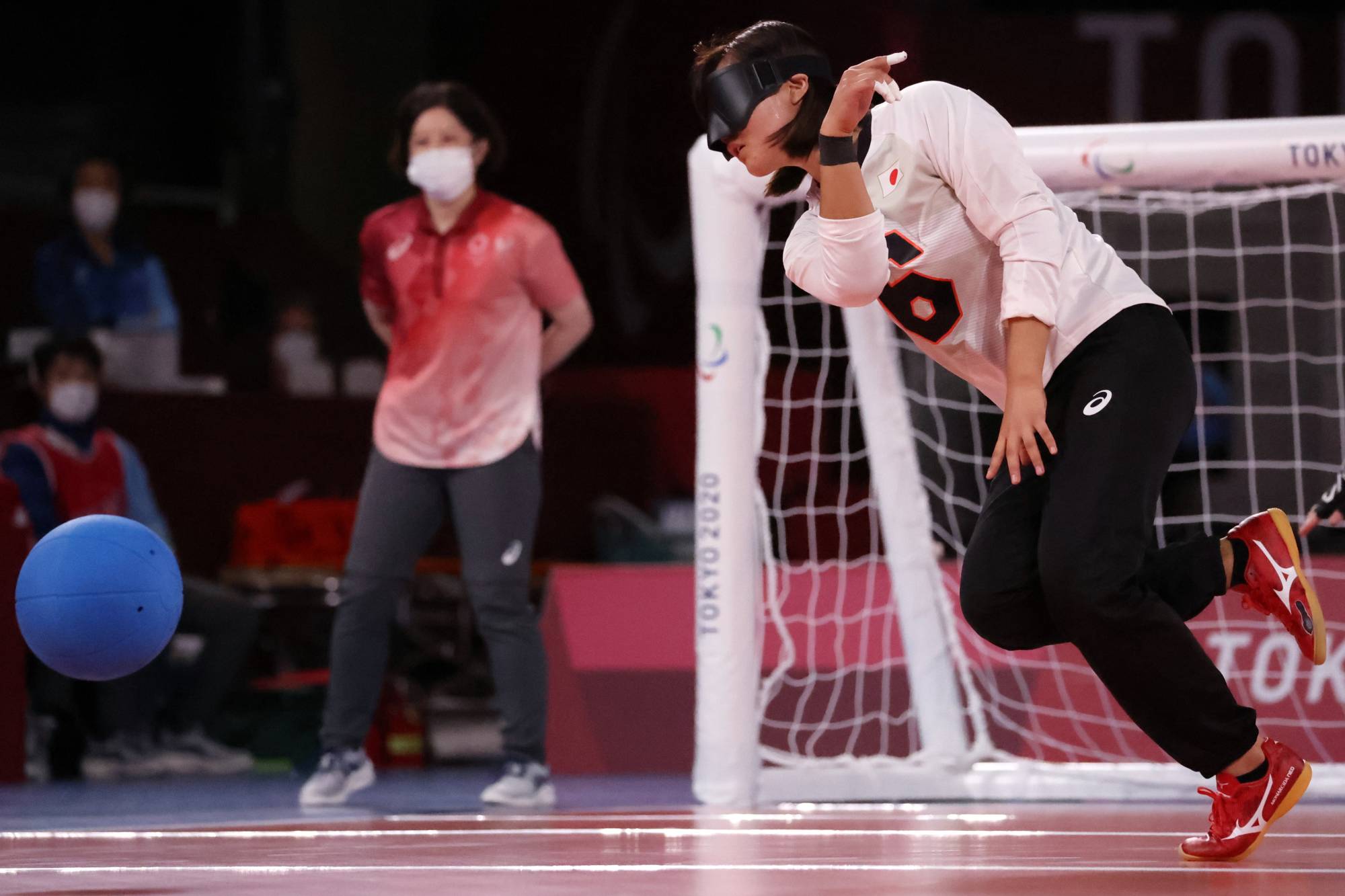In the image, a girl is seen engaging in a sport inside an auditorium, identifiable by the red floor with white lines and the gymnasium-like setting. The girl, wearing a black blindfold over her eyes, dons a white long-sleeve jersey displaying the black number 6, black pants, and red sneakers. She appears to be in motion, leaning forward as if she has just thrown or struck a blue ball, which is in midair to her left. In the background, a white goal net is visible, along with a few spectators who are all wearing white COVID masks. Additionally, another individual, wearing a red shirt, dark grey pants, and white sneakers, can be seen standing with hands behind their back near the goal net.